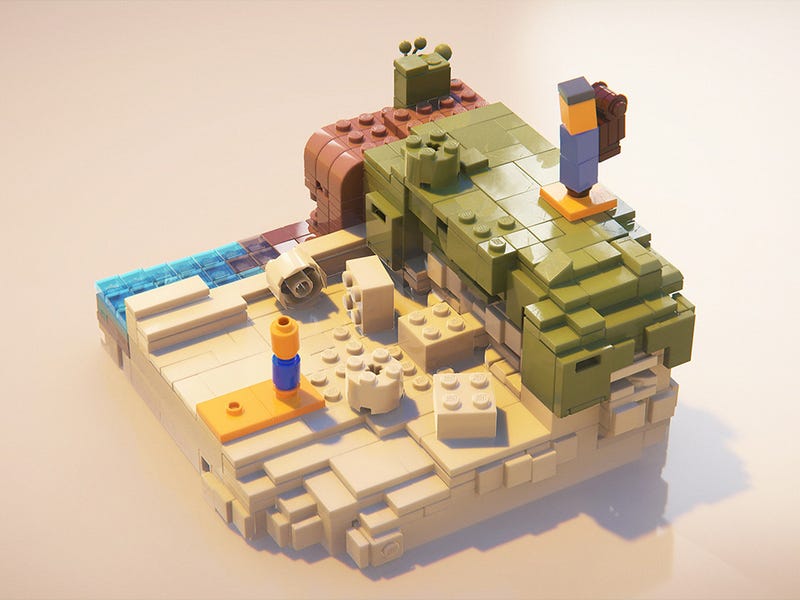The indoor, close-up, color photograph showcases an intricately assembled Lego creation on a clean, white base. The structure, predominantly rectangular and without a specific resemblance to any common object, features a variety of vibrant pieces meticulously put together. 

The bottom portion of the creation rests on a tan-ish white platform. Towards the back, there's an elevated, navy-green structure stretching upwards. The back-right area features a taller strip with distinct brown segments. In contrast, the front-left section of the structure is highlighted by squares in green and yellow shades, enhanced by the backlighting that casts shadows from top right to front left.

Moreover, the Lego assembly includes small characters, almost stylized in appearance. One character, placed on the tan base, consists of a purple circle topped with an orange piece, while another figure higher up comprises two purple squares forming the body, an orange head piece, and another purple square resembling a hat. This character also carries a brown backpack.

An additional distinctive figure in the model appears as a stick-like person, reminiscent of a small French fry, featuring a blue shirt, black topped head piece, and shoes, standing on a yellow Lego piece on the green terrain. This figure seems to interact with the environment, suggesting an intricate narrative within the Lego creation, perhaps looking down to a smaller figure without hair below, enhancing the mysterious and detailed nature of this imaginative construction.